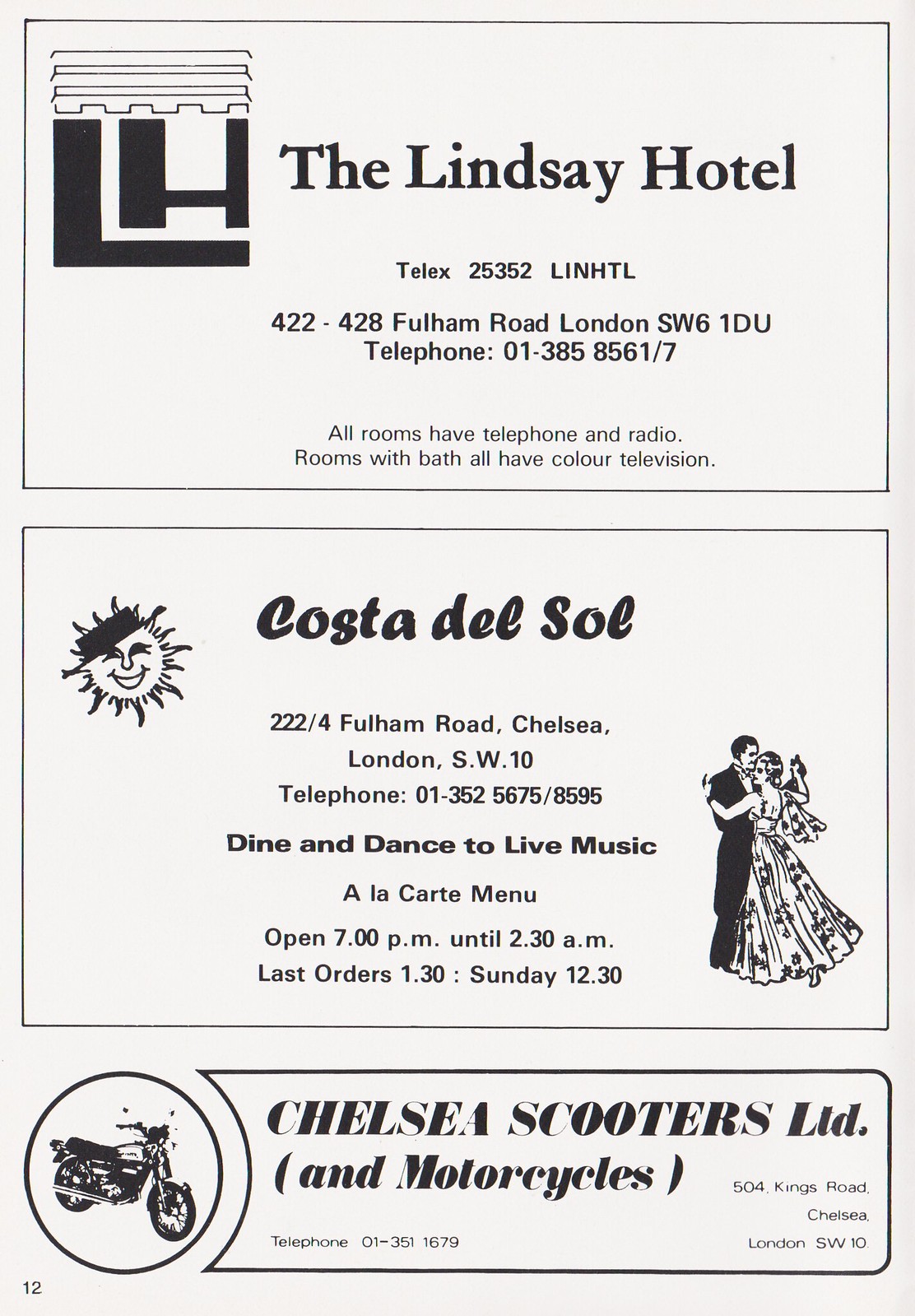This black-and-white rectangular poster features a light gray background and highlights three different businesses through distinct sections, each enclosed within its own rectangle. 

At the top, prominently positioned on the left side of the first rectangle, is a logo combining the letters "L" and "H," representing The Lindsay Hotel. To the right of the logo, specific details are listed: "The Lindsay Hotel, LX25352, LINHTL, 422-428 Fulham Road, London SW61D2, Telephone 013858561-7." The text also includes the hotel's amenities: "All rooms have telephone and radio, rooms with bath, all have color television."

The middle section features a drawing of a sun with a face on the left side, indicating the Costa Del Sol. On the right side of this box, an illustration of two people dancing accompanies the business details: "Costa del Sol, 222-4 Fulham Road, Chelsea, London SW10, Telephone 01352-5675-8595." Below this, the services are listed: "Dine and dance to live music, A La Carte Menu, Open 7.00pm until 2.30am, Last orders 1.30, Sunday 12.30."

The bottom section of the poster is dedicated to Chelsea Scooters, Ltd. On the left side, a circle encloses a drawing of a motorcycle. Adjacent to this illustration, the text reads, "Chelsea Scooters, Ltd, Bracket and Motorcycles, Bracket Close, 504 Kings Road, Chelsea, London SW10, Telephone 01351-1679."

Overall, the poster organizes and presents advertisements for The Lindsay Hotel, Costa Del Sol, and Chelsea Scooters, Ltd, each with specific logos, illustrations, addresses, contact information, and key service details.